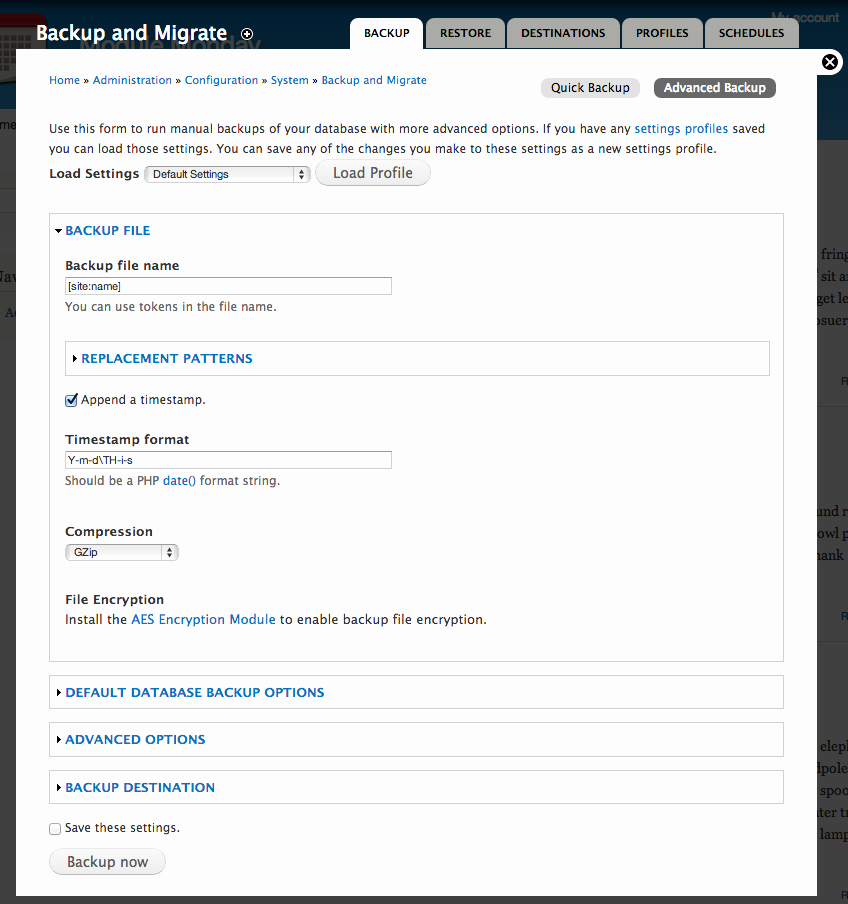In the top left corner, the title "Backup and Migrate" is prominently displayed. Adjacent to the right, there are menu options with a gray background: "Backup and Restore", "Destinations", and "Profiles and Schedules". Below these options, in the section labeled "Backup," there’s a detailed explanation: "Use this form to run manual backups of your database with more advanced options. If you have any settings profiles saved, you can load these settings. You can save any changes you make to these settings as a new settings profile."

Further down, highlighted in blue, is the label "Backup File" with a downward pointing arrow to the left. Under this label is the "Replacement Patterns" section, featuring a checkbox option labeled "Append a timestamp". Following this, there's another section titled "Compression" with a large rectangular input area beneath it. Next is "File Encryption," which advises to "install the AES encryption module to enable backup file encryption."

Below these options, in blue text, is "Default Database Backup Options", followed by "Advanced Options". The last selector is "Backup Destination". Finally, at the very bottom of the screen in very small text, there are two options: "Save These Settings" and the underlined "Backup Now".